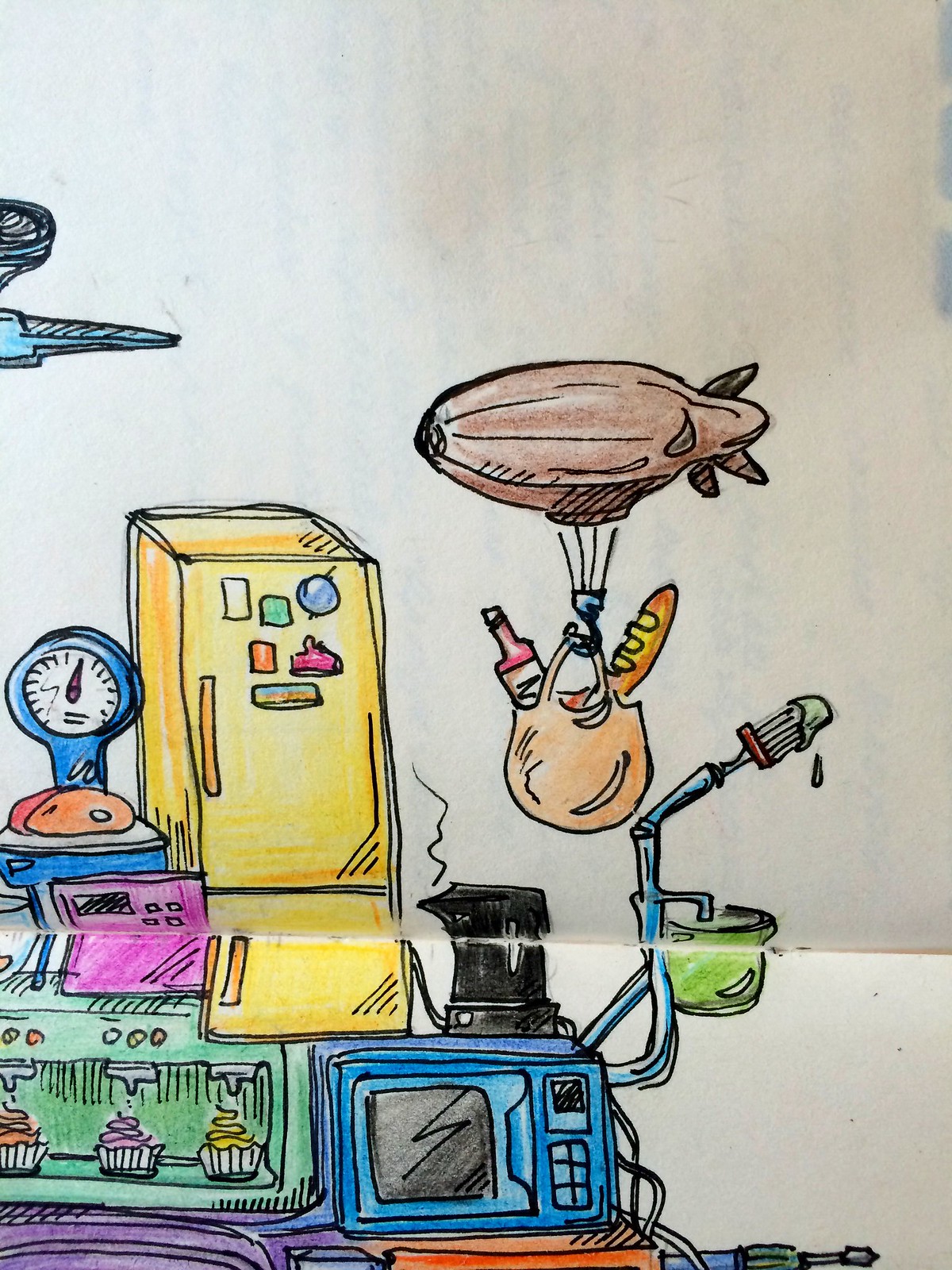This image showcases a highly creative and detailed sketch crafted in pen and ink, brought to life with colorful accents using colored pencils or possibly crayons. The artwork exudes a futuristic steampunk vibe, anchored by various intricately designed elements. Dominating the scene is a dirigible laden with a tote bag carrying bread and wine, floating majestically. Below, a small vintage computer shaded in blue is depicted, equipped with what appears to be either a microphone or an arm-like paintbrush, alongside a stylized glass with a spout.

Further adding to the intricate composition is a vertical, yellow-hued vintage computer tower-like structure, embellished with an array of knobs, dots, and lines that give it a face-like appearance. To its side, there is a dial with an analog pointer, enhancing the retro-futuristic aesthetic. In the lower left corner, a whimsical cupcake-making machine adds a touch of playful fantasy.

Above the computer, there is a kettle perched on a hot plate, hinting at a blend of old and new worlds. The upper left corner reveals the tail end of a flying machine, inviting the viewer's imagination to wander. The background is a textured canvas of stapled and folded paper, amplifying the raw creativity and handmade feel of this steampunk-inspired design.